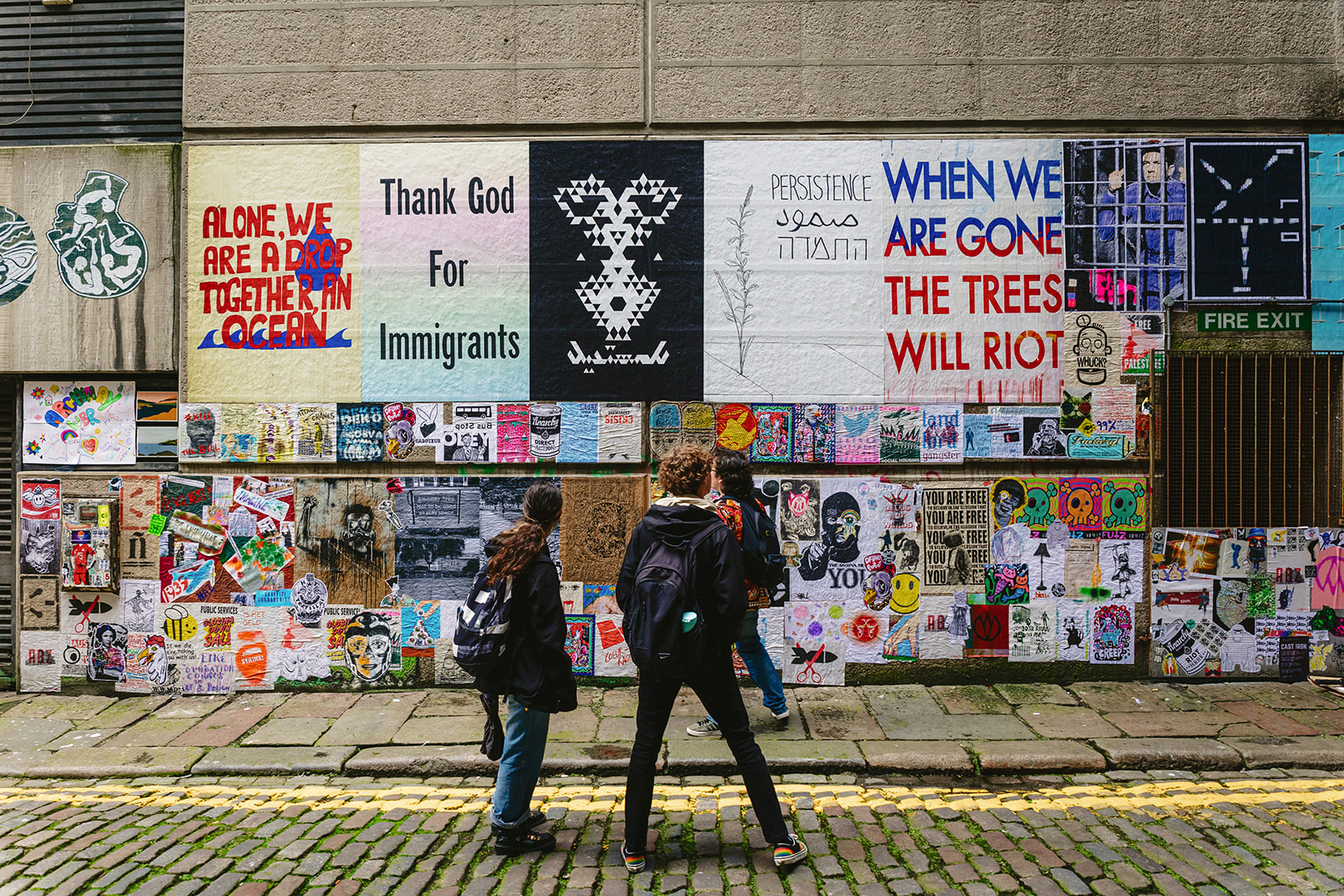The photograph captures an urban setting with a detailed scene of a graffiti-covered wall. The wall is adorned with various posters, murals, and political statements, including prominent texts such as "Thank God for Immigrants," "When We Are Gone the Trees Will Riot," "Alone We Are a Drop, Together an Ocean," and "Persistence." The artwork and posters are layered, with brighter, vibrant smaller images interspersed among larger, more prominent pieces. Near the top left corner of the wall, there’s a metal vent, and along its lower half, there is an illustration of a man behind prison bars.

In the foreground, three young adults stand on a cobblestone street, facing away from the camera, observing the wall. The sidewalk in front of the wall is made of large stone slabs, with light green moss growing between the cobblestones. The person on the left has long, wavy brown hair tied in a ponytail, wears blue jeans and a black jacket, and carries a backpack. The individual in the middle has short curly hair, dressed in all-black clothing with multicolored shoes and a backpack. The third person, partially obscured by the middle individual, wears an orange shirt, blue jeans, a black backpack, and has long black hair.

The scene captures a moment of quiet reflection among the three individuals as they engage with the dynamic and evocative street art before them.